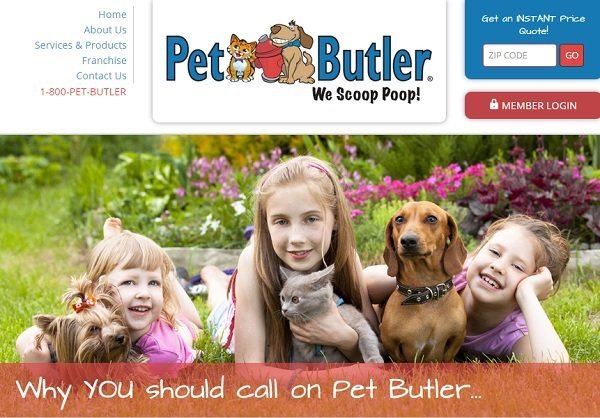This is a detailed screenshot of the PetButler website. The header, prominently positioned at the top center, is a white, rounded rectangle containing the website's logo. The logo features the words "PetButler" in blue, divided by a charming, cartoonish illustration of a cat and a dog hugging a garbage can. Below the logo, the tagline "We Scoop Poop" succinctly conveys the service offered. On the right side of the header, there's a feature to obtain an instant price quote, requiring users to enter their zip code in a text field. Adjacent to this is a red button labeled "Member Login." On the left side of the header, there are navigational links for "Home," "About Us," "Services and Products," "Franchise," and "Contact Us."

Dominating the main page is a photograph depicting three children lovingly holding their pets—two dogs and a cat. Notably, the cat appears displeased, characterized by its airplane ears. Superimposed at the bottom of the image is a translucent, reddish strip featuring white text. The caption reads, "Why You Should Call On PetButler," although the typography choice is notably poor.